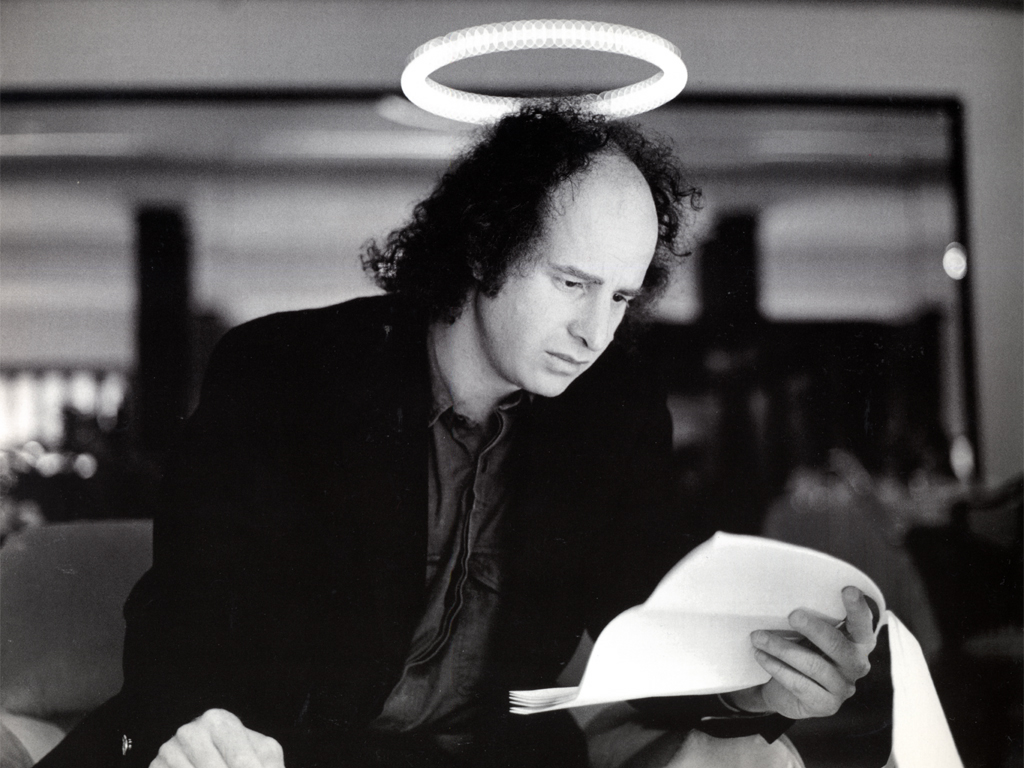The black and white image features Stephen Wright, the actor and comedian, who appears to be in his 30s or 40s. He has curly hair that reaches his shoulders but is significantly balding on the top of his head. Wright is wearing a dark sport coat over a dark button-up collared shirt. Seen from the torso up, he leans slightly forward, intently focused with a concerned expression as he looks down at a stapled group of white papers held in his left hand. His left arm rests on an armrest, and his right hand is placed on his leg. Adding a surreal touch, a circular light resembling a halo is above his head, likely a special effect. The background is blurred with indistinct black and gray objects, possibly including a window or wall.